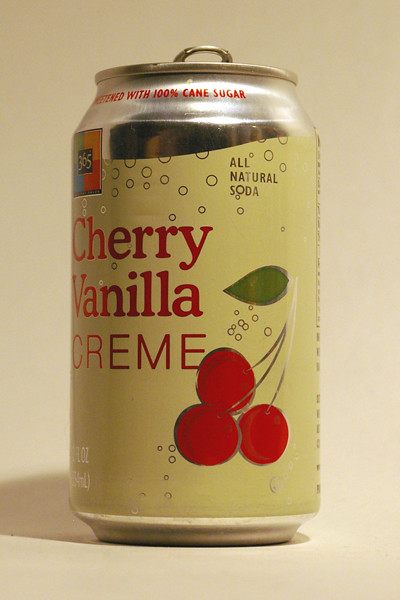This photograph features an aluminum can of soda with a metallic silver top and a label that transitions to a pale yellow color. The can, likely opened, has a visible pull-tab extending just above its top. Prominently displayed in dark and light red text on the front of the can, is the flavor description "cherry vanilla cream." The label includes an image of three bright red cherries with stems and a single green leaf, surrounded by illustrated bubbles to signify carbonation. 

Additionally, the can states "all-natural soda" and mentions that it is sweetened with 100% cane sugar. Also featured on the can is the Whole Foods 365 brand logo, depicted as a green, yellow, blue, and red checkerboard pattern with "365" in a small black square at the center. At the bottom of the can, some text indicating the fluid ounce weight is partially visible but cut off due to the curve of the can. The backdrop of the image is a light tan or pale beige color, with the can casting a shadow to the left.